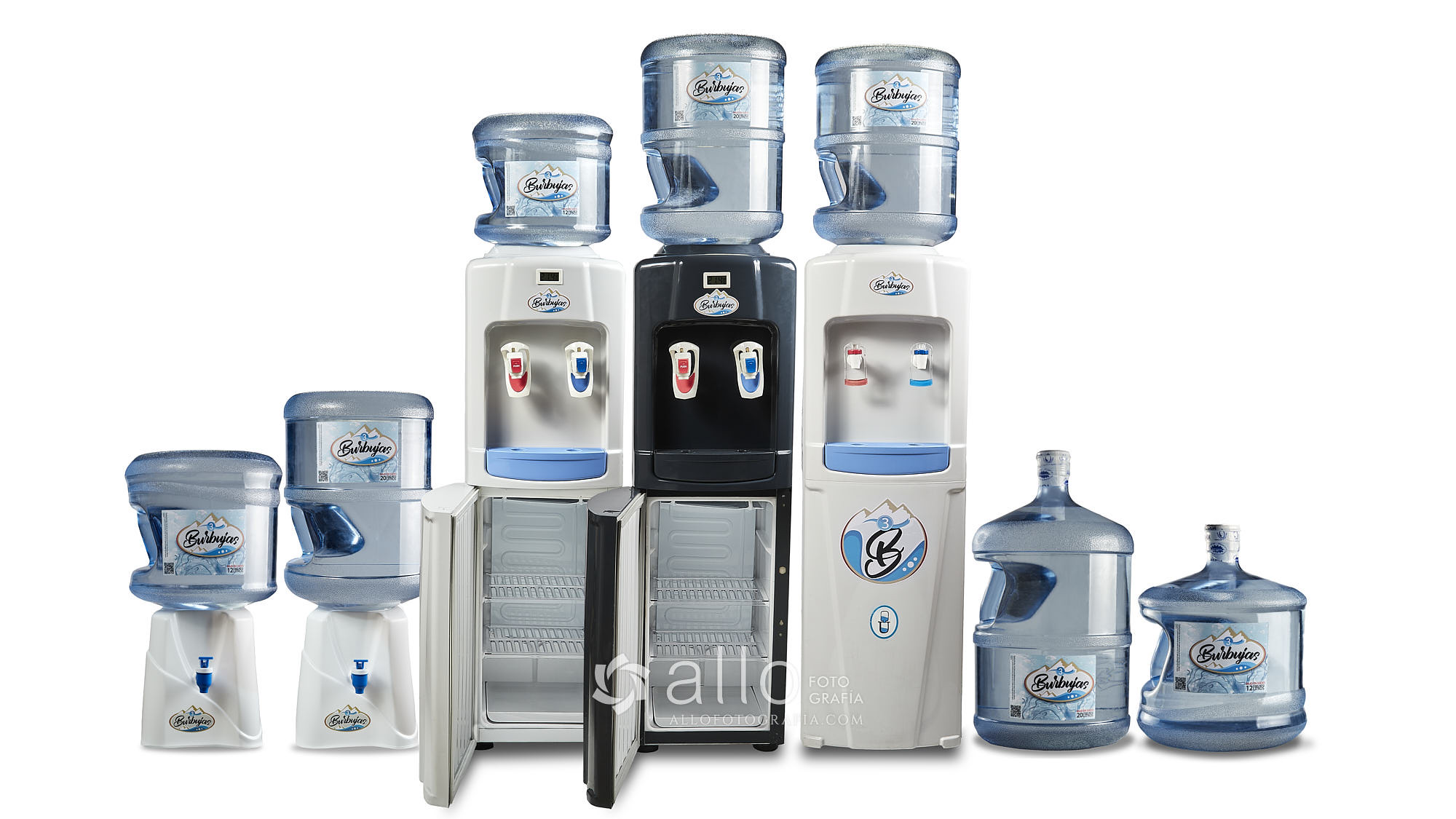This studio photograph, featuring a pure white background, showcases a lineup of various water dispensers alongside water bottles of different sizes. On the left side of the image, two shorter dispensers are positioned on a countertop, each with blue spouts: the one on the far left holds a smaller water bottle, and next to it, a slightly taller dispenser also supports a large bottle.

Moving to the center and right, three freestanding water dispensers are prominently displayed. Each unit is approximately three feet tall and equipped with both hot (red spout) and cold (blue spout) faucets. The dispenser on the left is white and has a mini-fridge at the bottom, which is shown with the door open, revealing two small racks inside. The middle dispenser is black, also featuring an open mini-fridge at the bottom with similar interior racks. The right dispenser is white as well but lacks a mini-fridge.

To the far right of these three freestanding units, two additional water bottles are placed on the floor. One of the bottles resembles a five-gallon jug, while the other is slightly smaller. This detailed setup provides a clear demonstration of the available dispenser and bottle options, likely aimed at helping viewers select the best fit for their hydration needs.